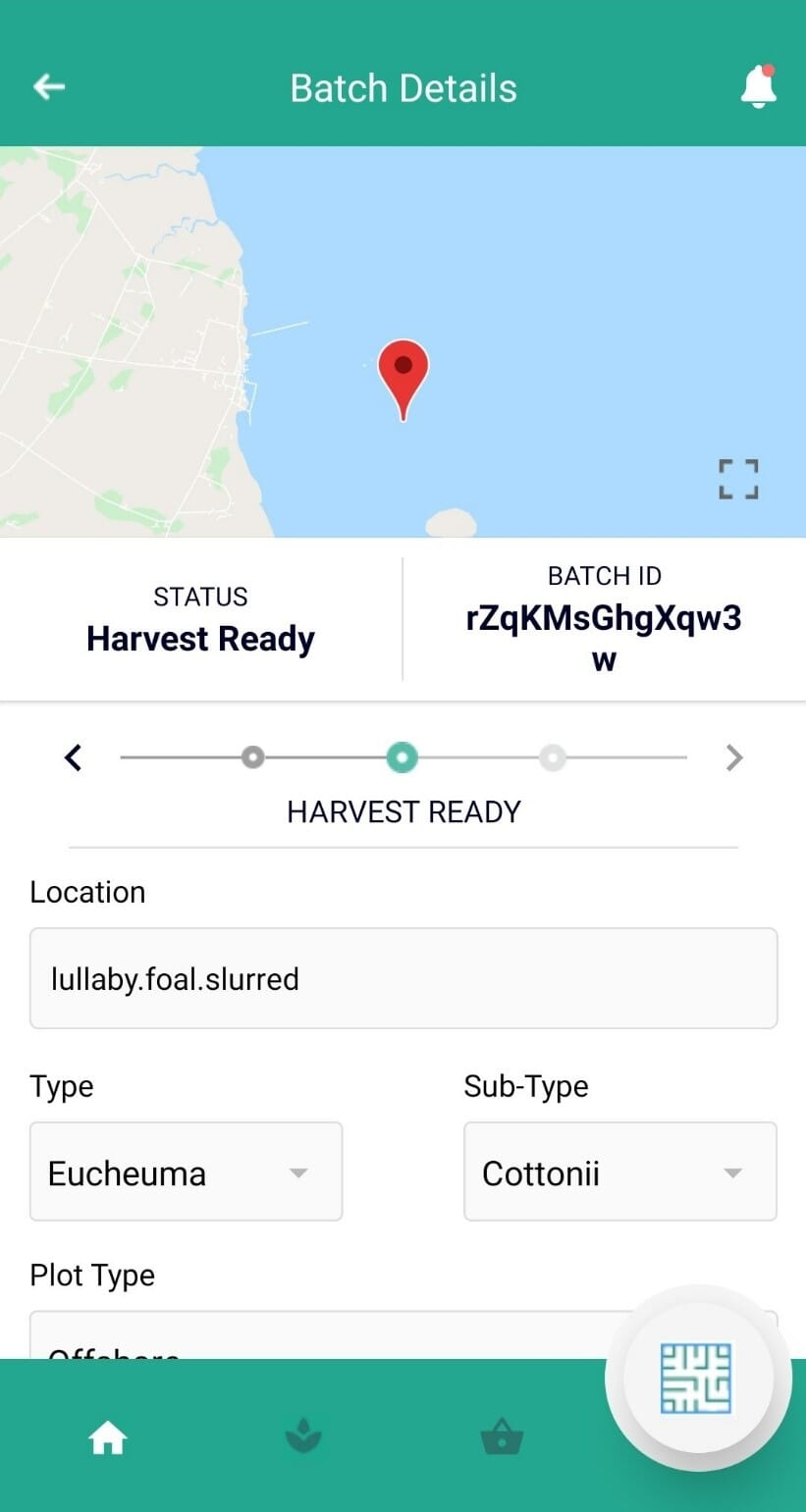A detailed screenshot showcases various elements pertinent to batch details. The central feature is a green bar displaying batch details in white text, accompanied by an arrow pointing left and a bell icon indicating a notification with a red dot. Below, a map with a location symbol—placed incongruously in the water—is visible.

To the right, a gray square box is presented. Key information detailed includes the status "Harvest Ready" and batch ID "RZQKMSGHXQW3W," reiterated by the phrase "Harvest Ready" multiple times throughout the image.

Three dots at the bottom provide visual status indicators, with the first dot in gray, the second in green, and the third in a very light gray. Additional data lists various locations and terms: "harvest ready, location, lullaby, dot FOAL, dot slurred; type of kahima: UCH, EU, MA; subtype: katoni: CO, TTO, NNI; plot type." An icon of a white house with a flower and basket is noted, alongside a green maze-like circle.

Overall, this richly detailed image captures essential batch information, location data, and visual status indicators critical for understanding the context of the batch being viewed.